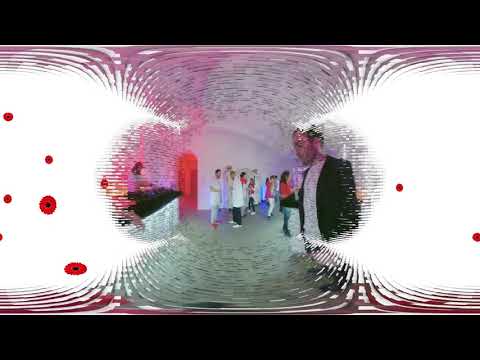The image depicts a heavily distorted interior setting with a central hourglass-like shape as the only clear part. It features multiple people standing inside a building with white walls, a white ceiling, and a light gray floor. Dominating the left and right sides are large white splotches with varying pink and purple stripes, interspersed with red dots - some containing black circles. In the far background, an arched doorway emits an orange light, adding a warm glow to the scene. On the left side, there is a white counter with a black countertop. Centrally, the image captures a group of people standing, possibly waiting or engaging in some sort of activity. Among them, near the right side, stands a man in a black sports jacket and white T-shirt, with short hair. The overall swirling and circular visual distortions imbue the image with a disorienting, surreal quality.